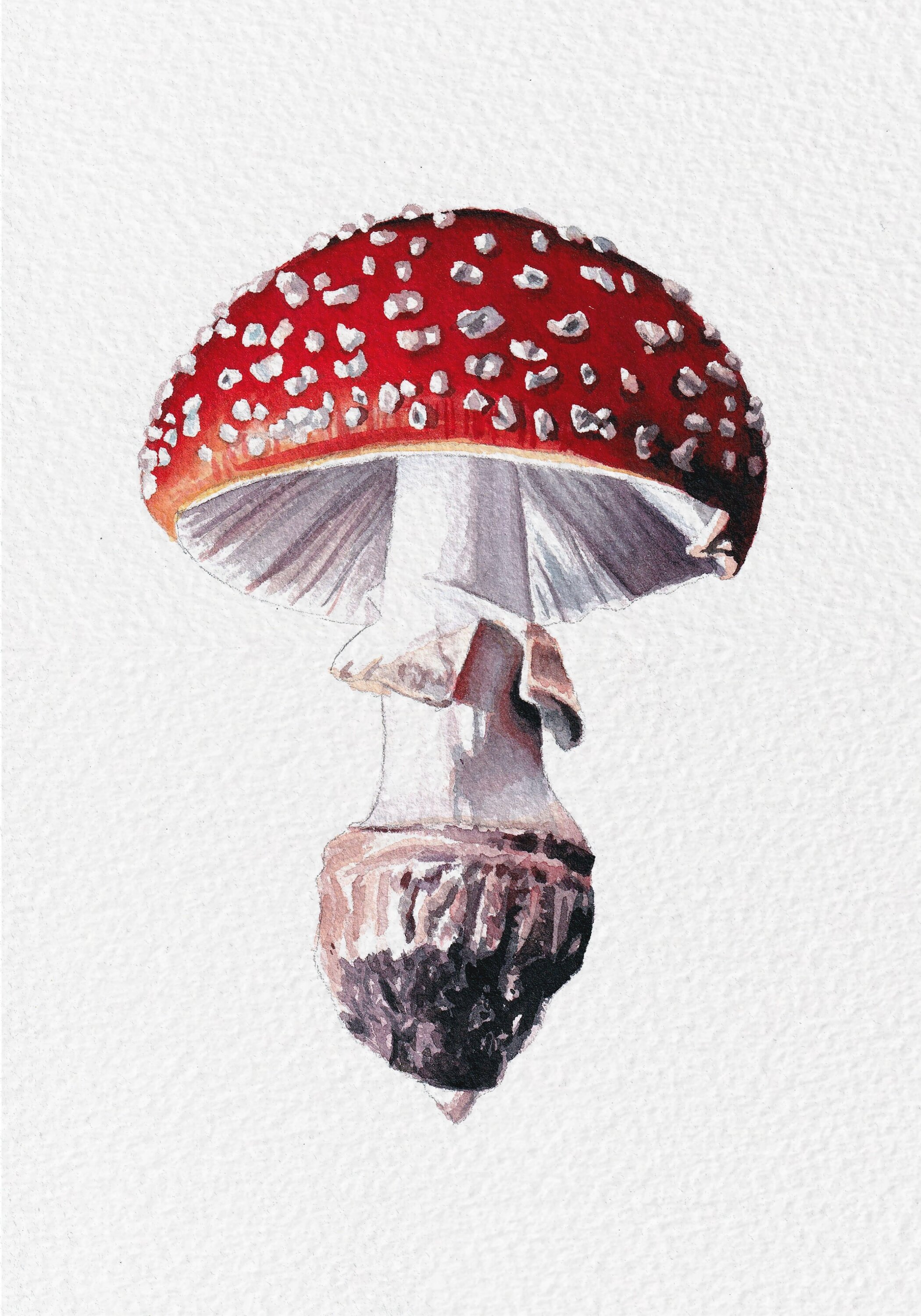This image depicts a highly detailed watercolor illustration of an Amanita mushroom on heavy-duty, textured white sketch paper. The mushroom’s vibrant red cap is adorned with numerous raised white specks, giving it a textured appearance. The underside of the cap reveals delicate grayish gills. The tall, white stalk features a rim or "skirt" about midway down, which varies in width. This stem descends into a tan, irregularly shaped base with visible black root-like structures, indicating where the mushroom was pulled from the ground. The backdrop is a light gray canvas that accentuates the rich colors and intricate details of the mushroom. There are no additional elements like text, people, or other objects in the image, focusing solely on the close-up of this beautifully rendered Amanita mushroom.